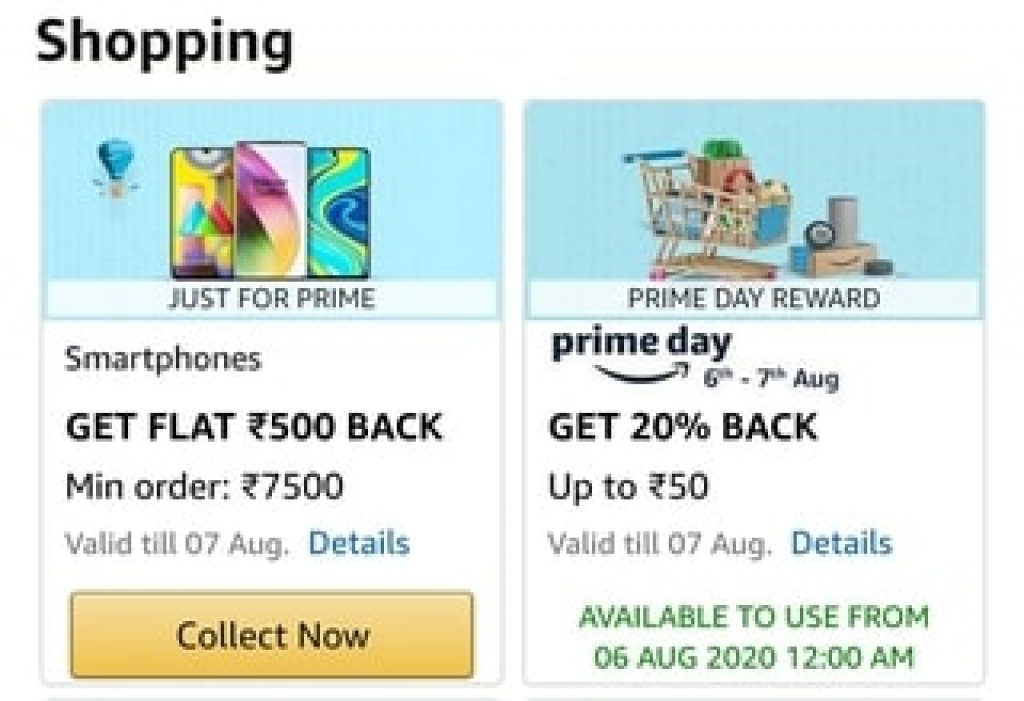The image showcases an Amazon promotional banner for Prime Day. At the top left, the word "Shopping" is prominently displayed in black text. The banner is divided into two sections, each promoting different offers.

On the right side, there's an image of a bronze or yellow shopping trolley filled with various items against a blue background. Below the trolley, text reads: "Prime Day Reward. Prime Day 6 to 7 August. Get 20% back up to 50 rupees. Valid till 7 August." Below this text, there is a blue button labeled "Details." Additional green text at the bottom states: "Available to use from 6 August 2020, 12 a.m."

On the left side, there is an image of three smartphones against a similar blue background. The accompanying text reads: "Just for Prime. Smartphones. Get flat 500 rupees back. Minimum order 7500 rupees. Valid till August." Underneath, a yellow button says "Collect now," and the text "Details" is in blue.

Overall, the banner effectively highlights exclusive Prime Day deals and rewards for Amazon members.